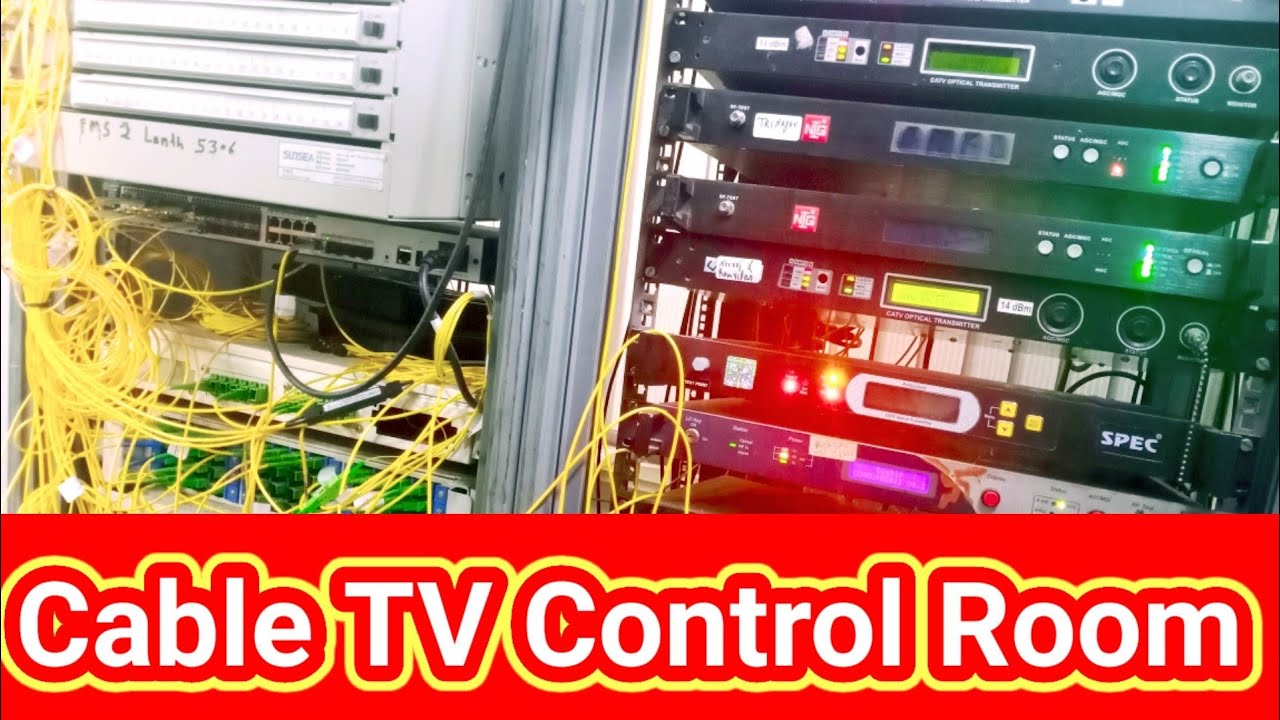The image features a Cable TV Control Room, prominently labeled at the bottom with bold, white text outlined in yellow on a red background, stating "CABLE TV CONTROL ROOM." The control room is a hive of activity, dominated by numerous yellow cables with green plugs, connecting to various control devices and electrical boxes. To the left, there's a gray device teeming with many yellow wires and green inputs. This equipment's screen displays "EMS 2 LENGTH 53.6," among other readings. To the right, stacks of black control units, each adorned with multiple buttons and lights, are visible. The top unit features a purple display, while the second unit has illuminated green LEDs. The black stack further includes a device marked "SPEC" in white lettering, accompanied by a plethora of cables, buttons, and connections, meticulously integrating the complex setup of the control room.